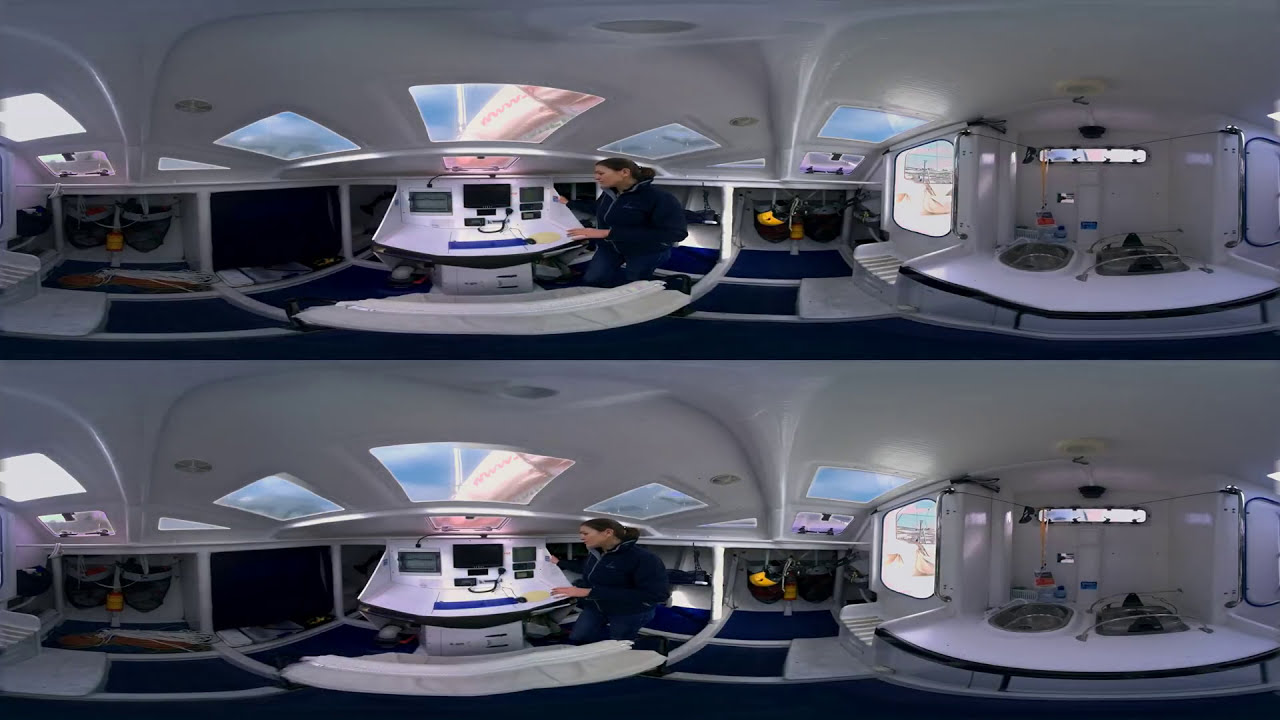This image presents a somewhat distorted panoramic interior view of a bright, white room, likely due to the use of a fisheye lens, which results in the top and bottom halves appearing identical. The room has white ceilings adorned with multiple skylights, through which the blue sky is visible. The walls are similarly white and feature several windows, making the space feel airy and well-lit. 

Dominating the scene is a woman with brown hair tied back in a ponytail, wearing a navy jacket and blue jeans. She is positioned near the center of the image, facing left (toward the nine o'clock position). She sits at a white table equipped with various rectangular objects, possibly control panels or screens. The table is flanked by built-in cabinets and cubbies.

To the right of the image, the room transitions into a kitchen area, identifiable by the white countertops and at least two stainless steel sinks. Above the countertops, beneath the cabinets, hang additional items, contributing to the room's functional appearance. 

This duplicity of the room's view, caused by the stacking of two panoramic images, gives the impression of an elongated, continuous space that encapsulates modern, possibly minimalist design elements, reminiscent of a mobile home or specialized work environment.